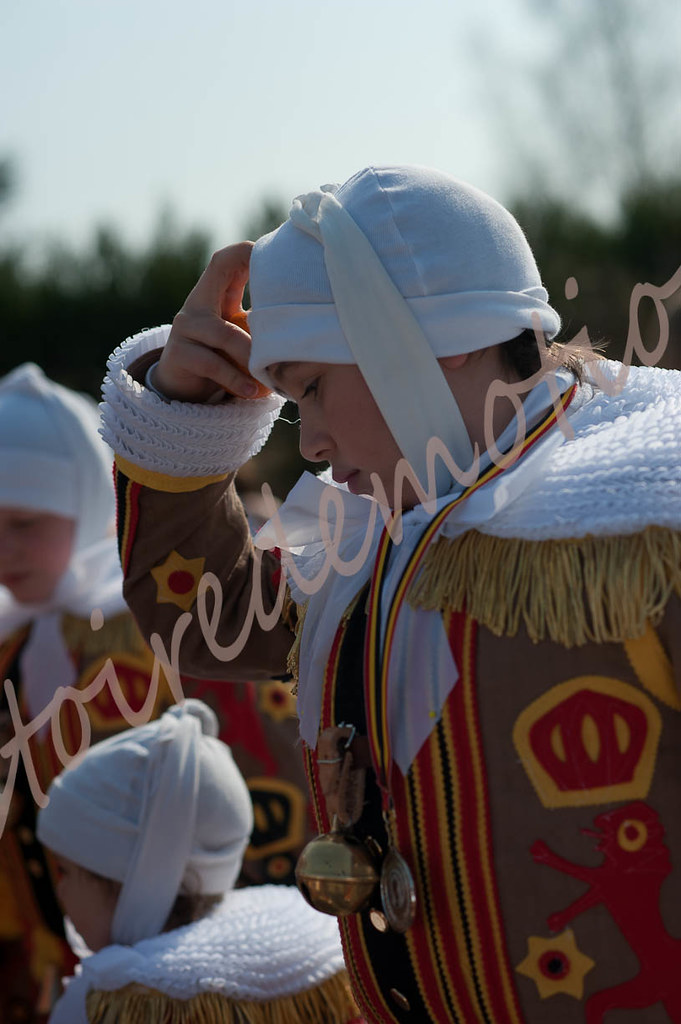This photograph captures a scene of a family dressed in elaborate winter attire, possibly participating in a cultural or religious ceremony. The individuals, including a young man, a young woman, and a little girl, are donned in thick, brightly colored costumes featuring shades of red, yellow, and brown. Each person wears a white hat or cap that covers their ears, with the man in the forefront securing his with a hand on his head. The man's outfit is adorned with metals around his neck, including a large bell. The girl's attire features intricate fringe and white crochet work on the shoulders and sleeves. The background is a blur of trees, suggesting a winter setting in what could be Central Asia. The scene is imbued with a festive or ceremonial atmosphere, underscored by the ornate and vibrant costumes.